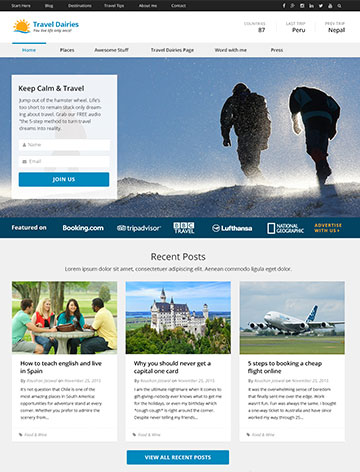This image appears to be a screenshot of a blurry travel website. At the top, there's a black bar featuring approximately six white submenu links. To the right of the black bar, there are several icons that appear to be social media icons, though their blurriness makes them hard to identify.

Below this bar, there's a white box with blue text that reads "Travel Diaries," accompanied by a small gold sun icon. It appears to list destinations such as Peru and Nepal, along with a price which is difficult to discern due to the blurriness.

Further down, there are more submenus, which seem to be about five or six in number. This section includes a white box that encourages visitors to "Keep Calm and Travel." There are two text fields, likely for entering a name and email address for more information, followed by a "Join Us" button in blue and white.

The main image depicts two people hiking through a snowy mountain landscape. Below this image, a blue bar contains the text: "Featured on Booking.com, TripAdvisor, BBC Travel, Lufthansa, National Geographic," along with a gold advertisement section.

Continuing down, there's a "Recent Posts" section with a brief sentence of text underneath. This is followed by a series of three images, each accompanied by black text. The first image shows a group of people sitting outside around a stone table during the day. The second image, which features a European-looking castle with a blue sky and green trees, includes text in a blue and white box that reads "View All Recent Posts." The final image shows a blue and white airplane.

Overall, while the blurriness makes some details difficult to interpret, the page clearly emphasizes travel destinations, recent posts, and encourages interaction through newsletter sign-ups and social media links.